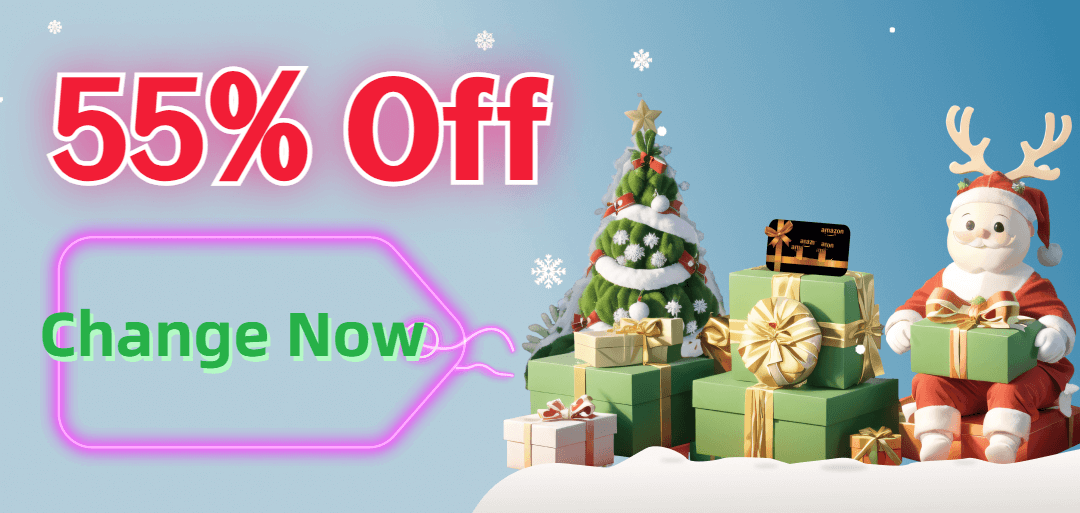Holiday Sale Advertisement: 

This festive, landscape-oriented image captures the spirit of the Christmas season with a blend of vibrant and playful elements. Dominating the scene is bold red text with a white outline proclaiming "55% OFF", next to an eye-catching pink neon price tag with green text and a light green shadow beneath it, urging viewers to "Change Now". 

A charming 3D Christmas tree, crafted to look like a stuffed toy, takes center stage. Surrounding the scene are delicate, floating snowflakes, enhancing the wintry feel. The background transitions from a light blue on the left to a darker blue on the right, giving a subtle yet pleasing gradient effect.

Scattered around the image are beautifully wrapped green gift boxes with ornate bows, adding to the holiday cheer. Among them is a black card placed atop one of the boxes, possibly a gift tag or a greeting card. On the right side, a stuffed Santa Claus figure adds a whimsical touch, adorned with a Santa hat that features reindeer ears on top. He holds a green gift box with a gold ribbon and bow on his lap.

At the bottom of the image, clusters of white, lumpy snow create the illusion that the scene might be set on a snowy rooftop, adding a curious and magical element to the composition.

Though the origin and specific purpose of the advertisement are unclear, it vividly conveys the theme of holiday sales and the joyful spirit of Christmas.